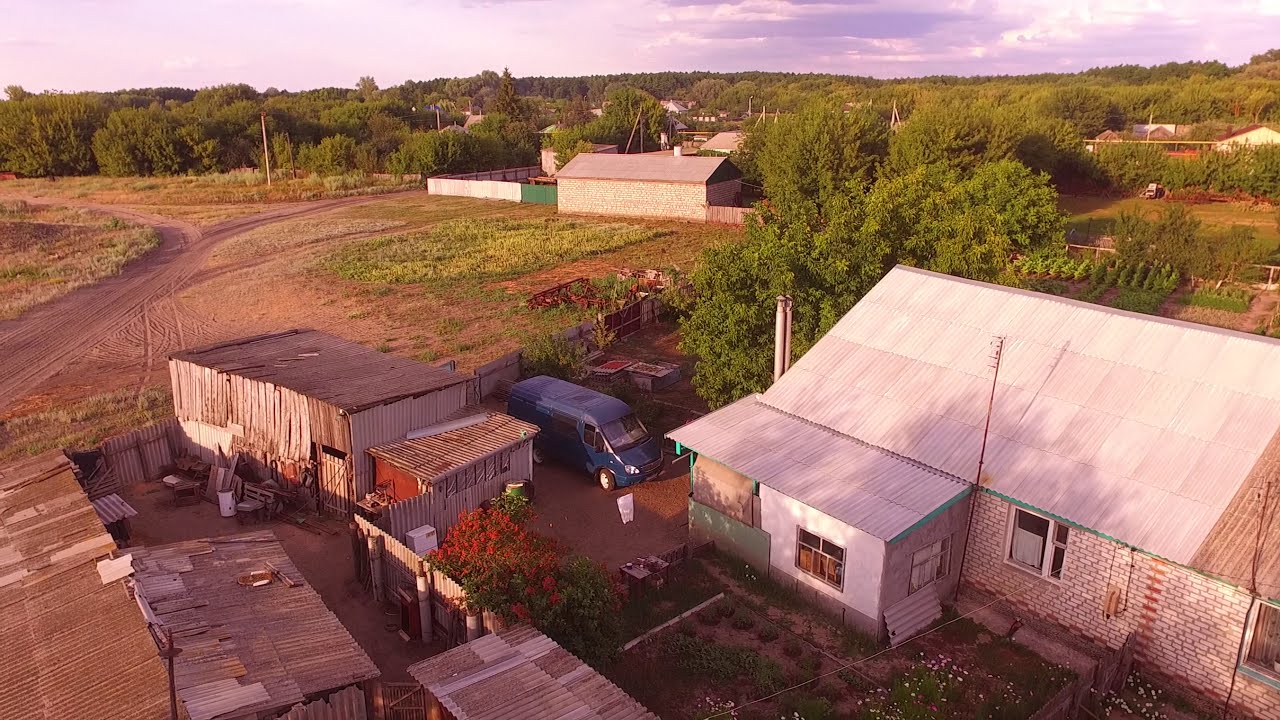The aerial image captures a rural farmland setting, likely taken from a drone at an angle during sunset, creating a reddish-purplish hue across the scene. The central focus is a dilapidated one-story white brick home with a slanted light gray tin roof, situated in the bottom right corner. In front of the house, there's a dark blue minivan parked near smaller structures that resemble sheds. Red flowers adorn the area around these sheds. Extending from left to right behind the van is a tall wooden fence, and further back, the property features gardens possibly growing vegetables. The dirt road with visible tire tracks leads up to the house from the center left of the image, winding towards the top left and center. Surrounding the buildings, numerous green trees add to the scenic landscape, while in the background, a few more brick houses and additional small structures are sparsely scattered. The sky is vivid with its blue expanse dotted by white clouds tinged with a purplish hue, adding to the overall tranquil and aged aura of the homestead.